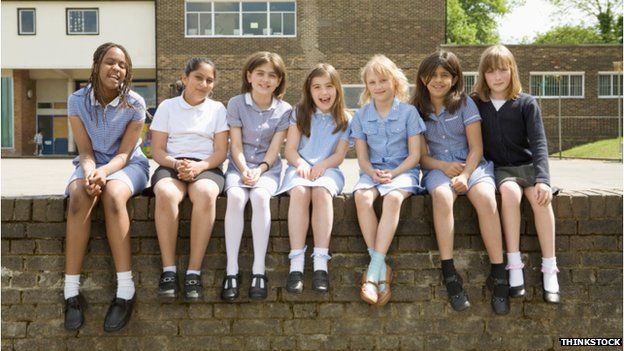The photograph captures a group of seven young girls, approximately aged between 11 and 13, sitting on a stone wall in front of a brown brick, two-story school building. The wall itself matches the aesthetic of the building, while fencing can be observed in the background. The girls are casually dressed in an assortment of colorful street clothes, including blue tops, white tops, a darker gray top, and white stockings. Their footwear varies, with most girls sporting black shoes and white socks, although one girl is seen wearing brown shoes and another with black socks. The girls have different skin tones and long hair, at least shoulder-length, reflecting the sunlight of what appears to be a sunny day. They are arranged in a line and are smiling, giving the impression that they are enjoying their time together.